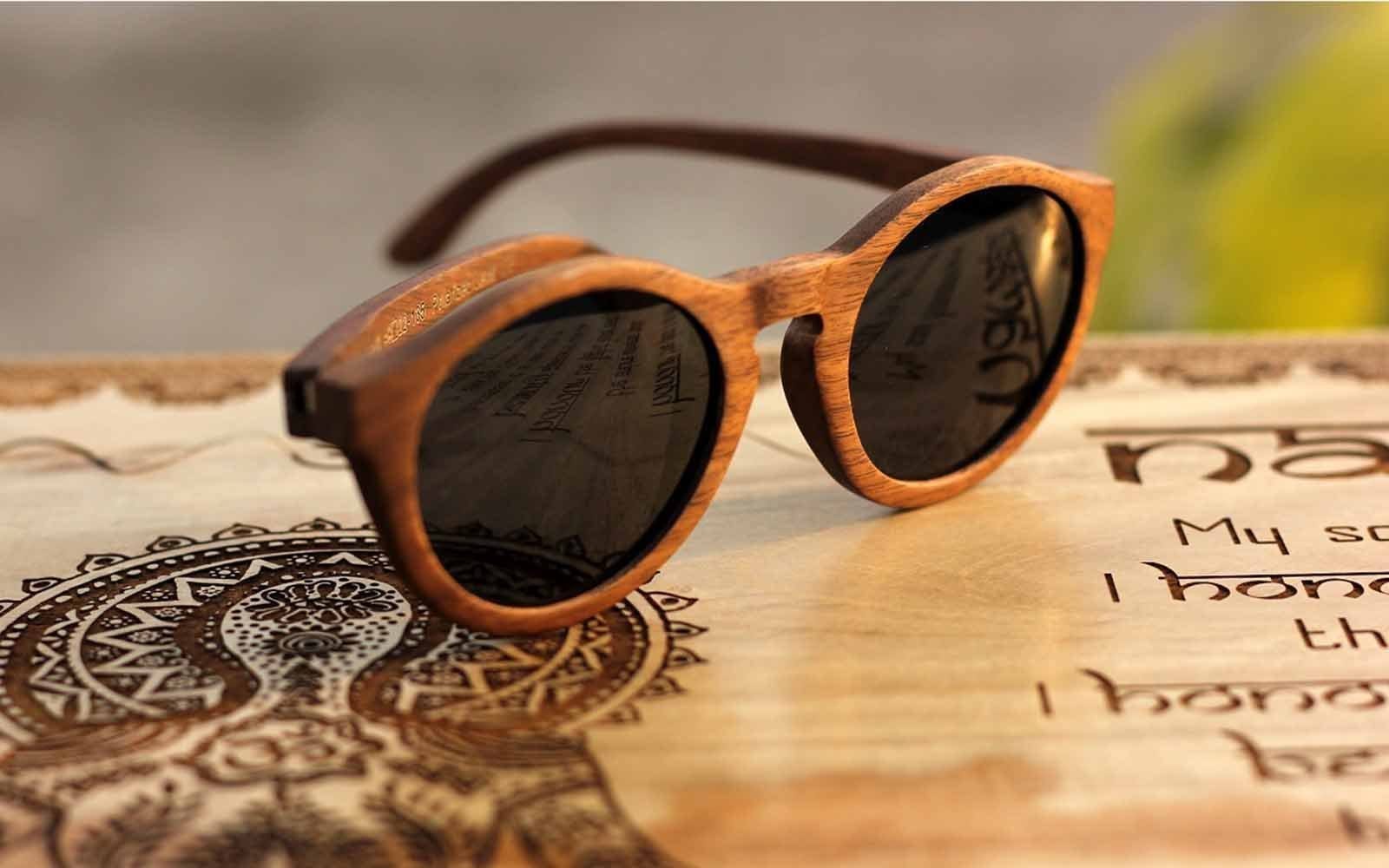The image showcases a pair of wooden sunglasses with dark lenses, resting on a brown board. The sunglasses are crafted from wood with a light to medium colored varnish, displaying a visible wood grain. One of the earpieces is open while the other is closed, causing the sunglasses to point towards the bottom right of the image. The dark lenses reflect the board's surface, which features intricate carvings and inscriptions.

The board itself has a textured appearance, with burnt or etched decorations, including the outline of a person surrounded by circular patterns, reminiscent of a rising sun behind the head, located at the bottom left corner. On the bottom right corner of the board, partially cut-off letters spell out "MY SONT H" but the complete words are unclear due to the reflection and angle. The background of the image is predominantly gray with patches of yellow and green visible in the upper right corner, adding to the overall ambiance of the scene. Light reflects off the board, making the inscriptions and carvings more prominent but still challenging to decipher fully.